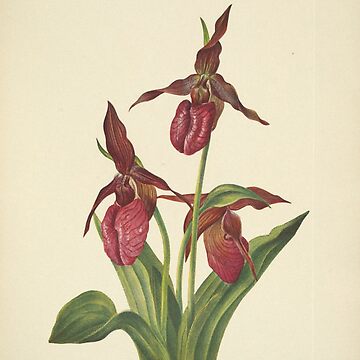This detailed illustration showcases a striking crimson red flower set against a pale, grayish pinkish-lilac background. The artwork, a nature-inspired painting, features three irregularly shaped flower sections, each perched atop long, thin, green stems. The distinctive blooms exhibit three prominent pointed petals stretching out like a three-pointed star, while a bulbous section with curling petals rests beneath them, resembling a lady slipper or even a glistening, veined human heart. Large, green leaves, reminiscent of corn husks, form a lush base, adding to the rich, textured composition of this unique botanical piece.